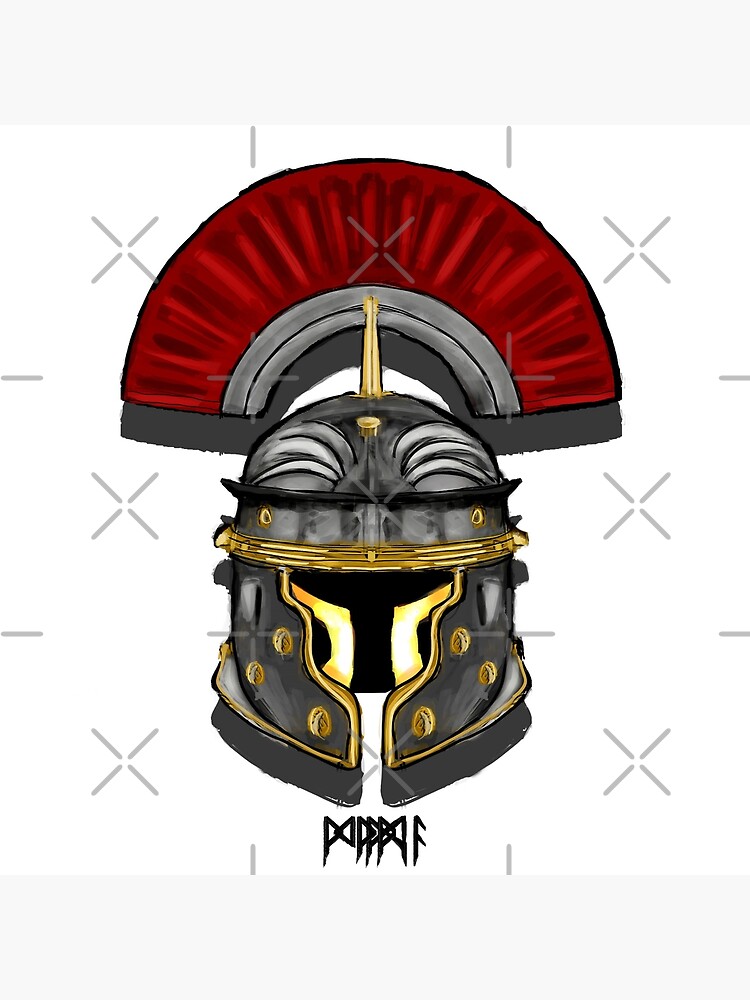The image depicts a detailed drawing of a knight's helmet, characterized by its grayish-black coloration and accented with gold. The helmet features a prominent, half-circle decorative crest at the top, which is red and resembles a fan or a rainbow arc. Below the crest, the helmet has a series of gold circles or rivets that add to its ornate design. The front of the helmet has a narrow opening that would provide visibility for the wearer's eyes, nose, and a small part of the mouth, suggesting it’s designed for functionality as well as aesthetics. The image is set against a white background and includes some lettering underneath the helmet, which appears as non-English symbols or runes, possibly the artist's signature or a decorative touch. Throughout the image, there are repeated instances of X's and dashes overlaying the helmet, potentially indicating a watermark or a copyright symbol.